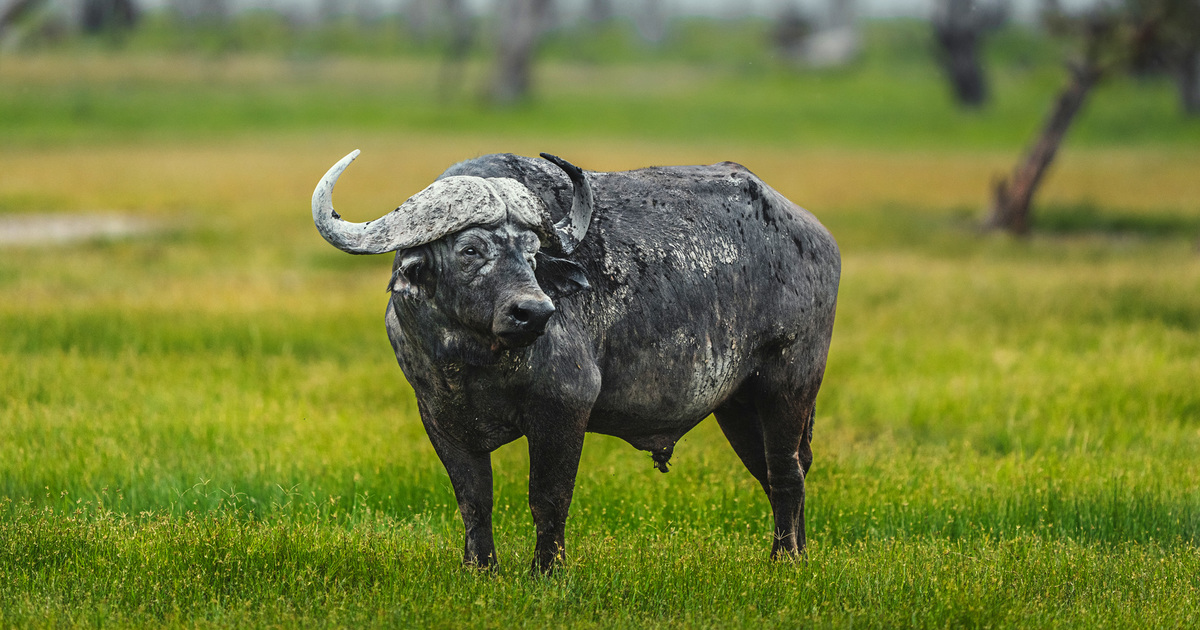This is a daytime outdoor photograph capturing a black ox standing in a lush green field. The ox, potentially a female given the faint visibility of an udder, commands the center of the image with its head slightly turned to the left, looking away from the camera. Its body exhibits distinct white markings amidst the black fur, and it has large, grayish-white horns that extend sideways before curving upwards. The grass in the foreground is vibrant and green, while the mid-ground reveals patches of brownish grass and a discernible tree trunk or branch to the right. The background is intentionally blurred, revealing indistinct but recognizable trees and more green grass, enhancing the depth of the scene. The texture of the ox has a rugged appearance, almost statue-like, adding an intriguing element to the overall composition.